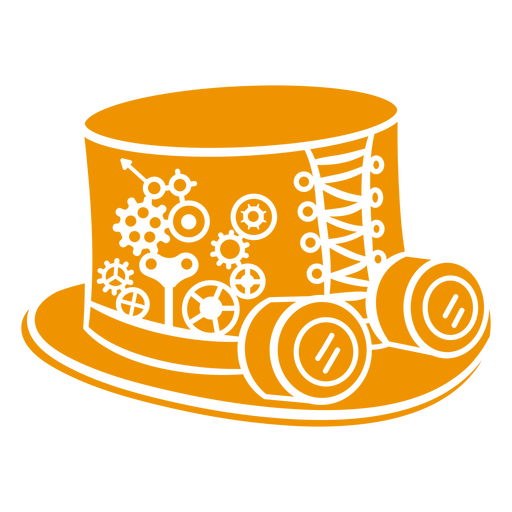The image depicts an intricately designed, orange and white top hat with various detailed decorations. The hat features a white-trimmed brim adorned with two cylindrical shapes that resemble binocular lenses. A string of zigzag laces, similar to shoelaces, runs up the front, flanked by vertical lines and small circles. On the side of the hat are interconnected round gears and an old-fashioned key, suggesting a steampunk aesthetic. Additionally, an arrow points upwards from these gears, and the hat includes a band around the brim. The illustration, likely created using digital tools like Illustrator or Photoshop, evokes the appearance of a ring leader's hat with a scientific, gadget-filled twist.